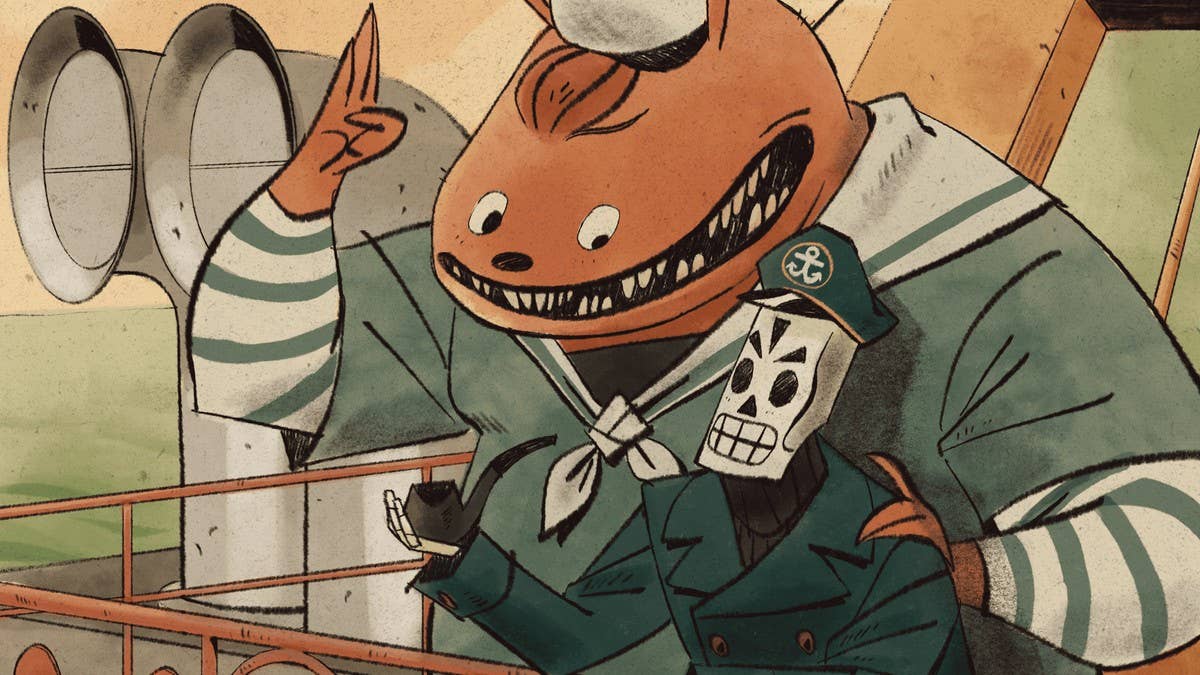This detailed illustration, appearing as a vibrant and somewhat eerie cartoon panel, depicts a scene on a ship featuring two distinct characters amidst a backdrop of nautical elements. The larger figure is an enormous, orange-furred creature with a round, brown head and a tuft of rust-colored hair. His face is wide with an exaggerated grin full of sharp, white teeth, giving a menacing yet oddly friendly appearance. He wears a green sailor shirt with a white sailor collar adorned with green stripes and a white and green neckerchief. His right arm is raised in a partial salute, revealing sleeves from an underlying white shirt with green stripes.

Standing in front of him is a smaller, skeletal figure with a rectangular skull-like face, black eyes, and a triangular nose hole. This character, presumed to be the captain, is dressed in an emerald green captain's coat buttoned with gold and a captain's hat bearing a white anchor emblem. He clutches a black pipe in his right hand and has a grimacing expression.

The background sets the scene on a ship, with visible teal-colored water indicating waves. There are red guardrails and two large, silver pipes resembling smokestacks on the left, adding to the maritime ambiance. The overall color palette features oranges, blues, and grays, enhancing the illustration's contrasting tones and creating a vivid, captivating maritime tableau.